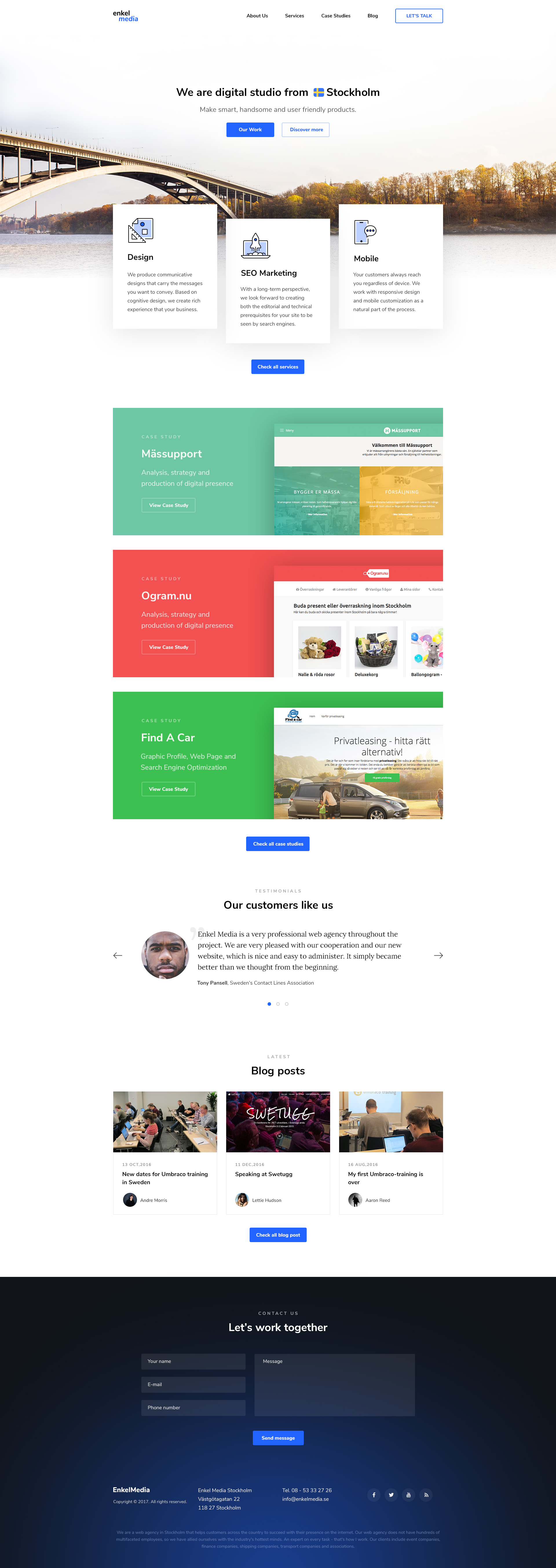Screenshot Description:

In the image, we see a screenshot of a webpage from a company named "Ankle Media," located in the upper left corner. To the right of the company name are navigation links labeled "About Us," "Services," "Case Studies," "Blog," and a call-to-action button that reads "Let's Talk."

Below the navigation bar, a vibrant color photograph depicts a serene river flanked by lush trees. The tree line runs horizontally across the image, and a bridge extends into view from the left side. Above the scene, a grayish-blue sky serves as the backdrop for a bold statement: "We are Digital Studio from Stockholm. Make smart, handsome, and user-friendly products." 

Two call-to-action buttons are positioned beneath this text — the first one on the left, colored blue, is labeled "Our Work," and the second one on the right reads "Discover More."

The bottom section of the page has a dark bluish-black background. Here, we find contact options with the headings "Contact Us" and "Let's Work Together." A form prompts the user to enter their name, email, and phone number, along with a message. Directly beneath the form is a blue action button labeled "Send Message."